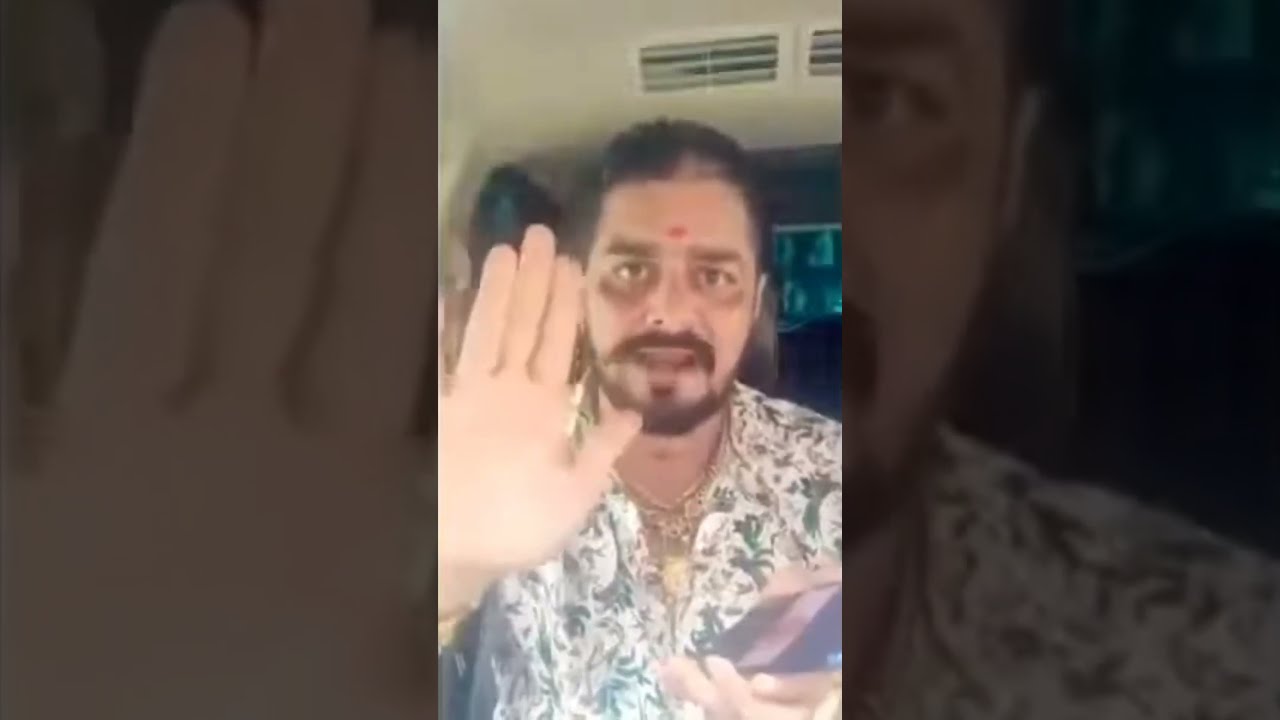The image appears to be a thumbnail for a YouTube or social media video featuring a man who looks to be of Indian descent, aged between 30 and 40. He has a beard, mustache, long hair tied back, and a red dot on his forehead. He is dressed in a stylish white and blue Hawaiian shirt with leafy designs and wears several gold chains around his neck, along with a gold watch. The man is seated inside a tan-roofed car, possibly in the back seat, featuring blue-grey upholstery and tan air vents above his head. He is photographed in mid-speech, directly engaging with the camera while raising his right hand. The main image is supplemented by two additional photos on either side: the left photo highlights his raised hand, while the right photo provides a side view of his face. His left hand seems to be holding an object, possibly a credit card. There are noticeable bruises under his eyes, suggesting injury.